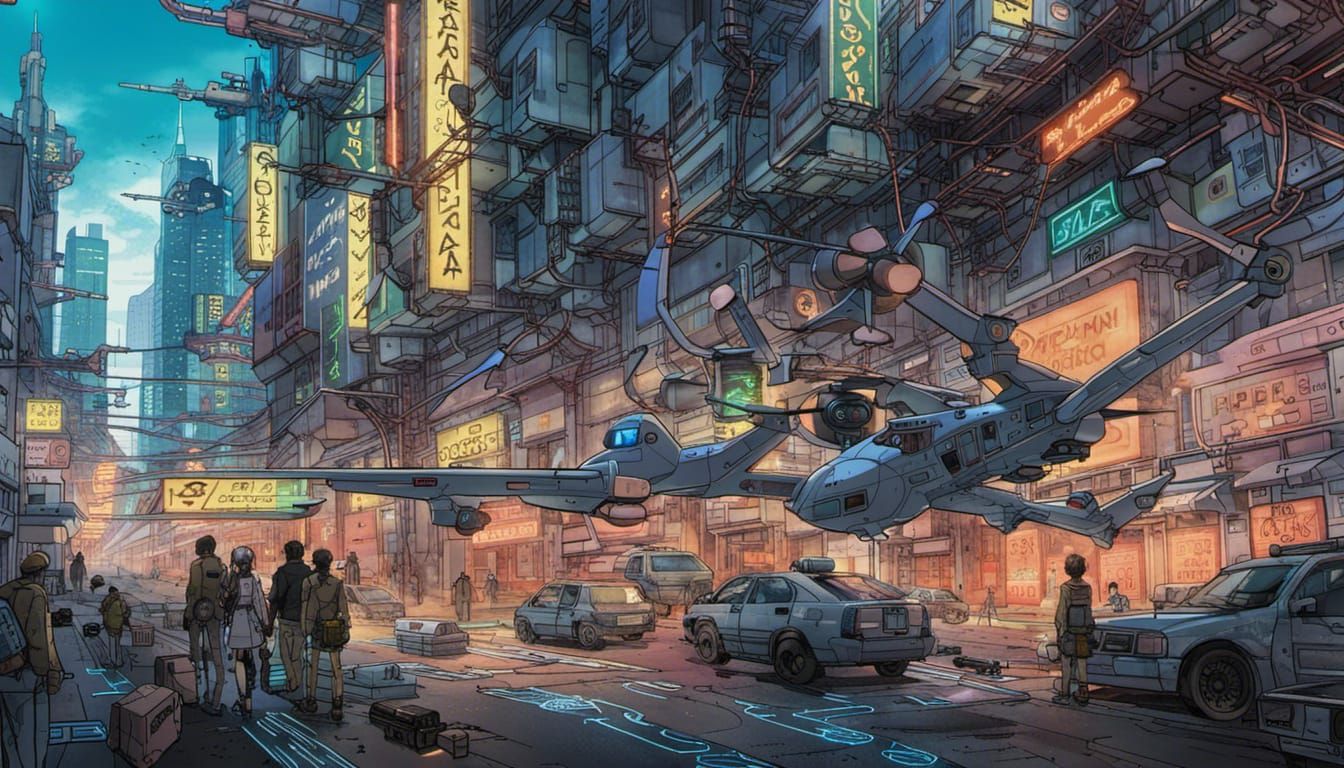This detailed cartoon drawing of a futuristic cityscape, reminiscent of an anime or a scene from Blade Runner, is presented in a horizontal rectangular format, about twice as wide as it is tall, measuring approximately six inches wide by three inches high. The scene is set in the middle of a towering, high-rise city with distinctive tall buildings adorned with vertical neon signs, possibly in foreign scripts such as Arabic or Asian languages like Japanese or Chinese. These signs contribute to the bustling atmosphere of the city.

In the foreground, the street is a highlight with its grid-like pattern illuminated in blue. On the left side, there are people walking, appearing somewhat confused, while on the right, there are parked and possibly wrecked vehicles. The street is cluttered with various objects like TVs and boxes, possibly debris from an earlier disturbance. Above the street, several gray hybrids, blending features of helicopters and airplanes—potentially drones—fly low over the scene.

The upper left-hand corner of the image features a blue sky with clouds, though the overall ambiance suggests it is either night or evening, as darkness pervades the scene with brightly lit buildings providing contrasting illumination. This detailed piece of art captures a chaotic and intriguing urban environment, blending futuristic themes with a sense of turmoil and complexity.